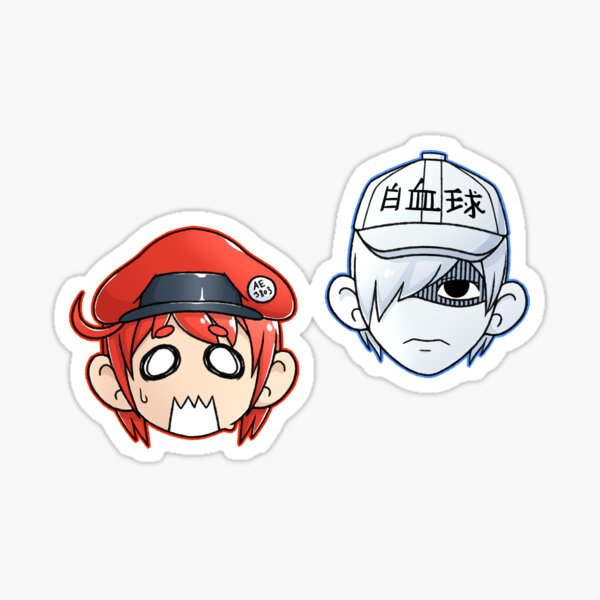The image portrays two chibi-style anime characters on a white background, each outlined in gray. The character on the left has vivid red hair and wears a layered combination of hats—a red beret over a black cap. This character's notable features include large ears, round white eyes without pupils, and a torn-like, jagged mouth with black rings around the eyes, giving a peculiar and slightly eerie appearance. The character on the right, outlined in blue, wears a white baseball cap adorned with Japanese characters. This character has light-colored hair that partially conceals a striped mask covering one eye, while the other eye remains visible. Distinctive features include large ears, an absence of a nose, and a minimalistic two-line mouth. Both characters appear to be stickers, likely merchandise from the anime "Hataraku Saibō" (Cells at Work!), popularly recognized as white blood cell representations.